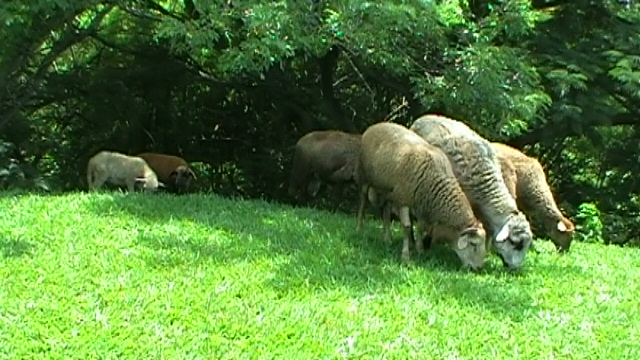In this vivid outdoor photograph, a herd of sheep grazes on a lush, bright green grassy field. The tall blades of grass sparkle under abundant yellow sunlight, interspersed with shadows cast by trees overhead. On the right-hand side of the image, three sheep stand side by side, their heads down as they munch on the green grass. These sheep have fluffy white coats with tinges of brown. In the background, two more sheep, one white and one brown, also feed on the grass, their forms partially concealed by the rich, green foliage. The backdrop features densely packed trees with dark trunks and a thick canopy of green leaves, adding to the natural setting's woodland ambiance. Scattered throughout the scene are shafts of sunlight filtering through the trees, highlighting the pastoral tranquility.